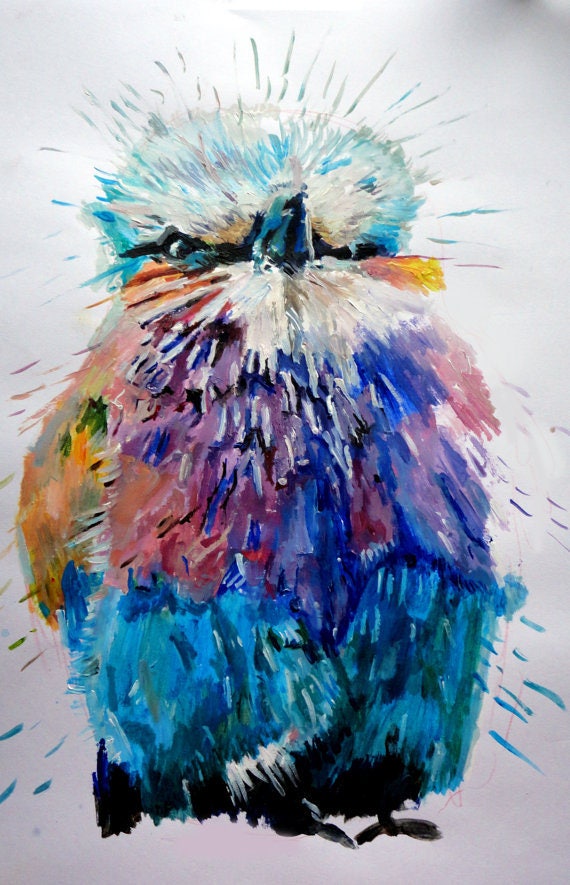This image portrays a beautifully detailed, impressionistic watercolor painting of a colorful bird viewed from the front. The bird, appearing fluffy and somewhat rotund, stands on its black feet, directly facing the viewer with a small beak and expressive eyes. Its predominantly white head contrasts vividly with bright aqua blue accents. The bird's shaded body showcases an array of vibrant hues: the upper parts in rich purples, bright and dark blues, with splashes of orange, green, and peach on its wings, and a touch of yellow tuft under its right eye.

Notably, there's an effect of dynamic movement, as if the bird is shaking and dispersing the colors into splashes around it. Bold, expressive brush strokes fill the composition, giving it an abstract and energetic quality. The painting's background gradient slightly shifts from a light grayish blue at the top to a light grayish pink near the bottom, enhancing the vividness of the bird. The overall piece is vertically oriented, adding to the portrait-like impact of this striking and colorful avian subject.